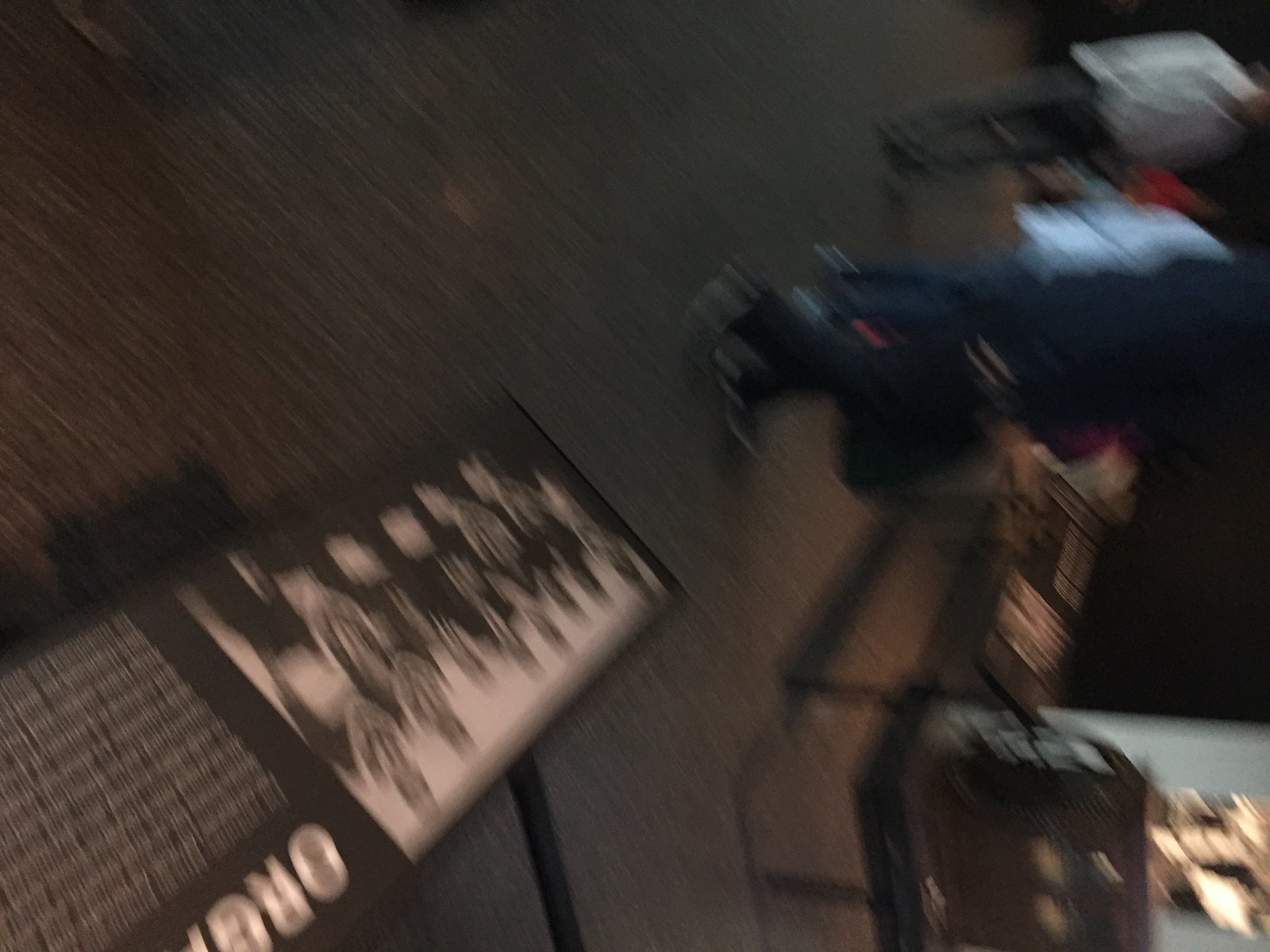This blurry photograph, taken with the camera rotated 90 degrees to the right, features several interesting elements. In the bottom left corner, protruding into the frame, there is a sign with some white text on it. The sign appears to have images of people on it, though they are not clearly visible. Towards the right side of the image, near the center, three indistinct figures are walking by. The person in the front is wearing a navy blue sweatshirt and black pants.